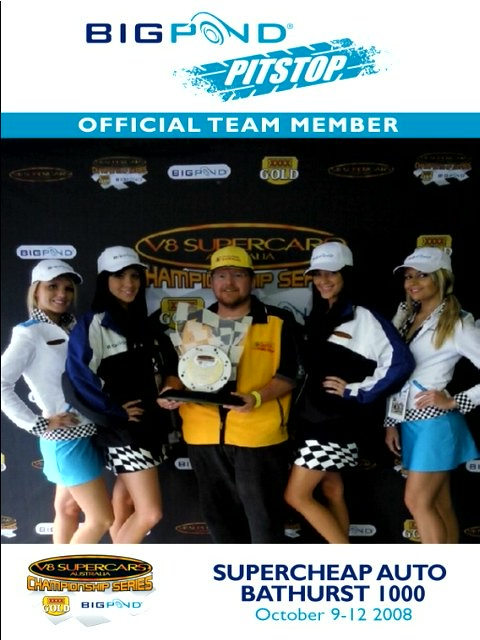In this photograph taken at a winner's circle event, a man stands proudly at the center, holding a trophy with a circular top and a black base. He is dressed in a large yellow and black jacket, a yellow cap, and black pants. On either side of him are four women, each of them smiling. The women on the left, one with brown hair and one with blonde hair, are dressed in short skirts with a black and white checkered flag design. Their white hats and jackets with blue stripes complement their outfits. The women on the right, one with brown hair and one with black hair, are wearing blue skirts and white blouses, which also feature the black and white checkered pattern on the waist, cuffs, and collar. Behind them is a black banner displaying the text "Big Pond Pit Stop official team member" in white and blue lettering. Advertisements cover the background, and at the bottom of the banner, it reads, "Super Cheap Auto Bathurst 1000, October 9-12, 2008," and "V8 Supercar Championship Series Gold, Big Pond." The group's coordinated attire and cheerful demeanor capture the celebratory spirit of this championship moment.